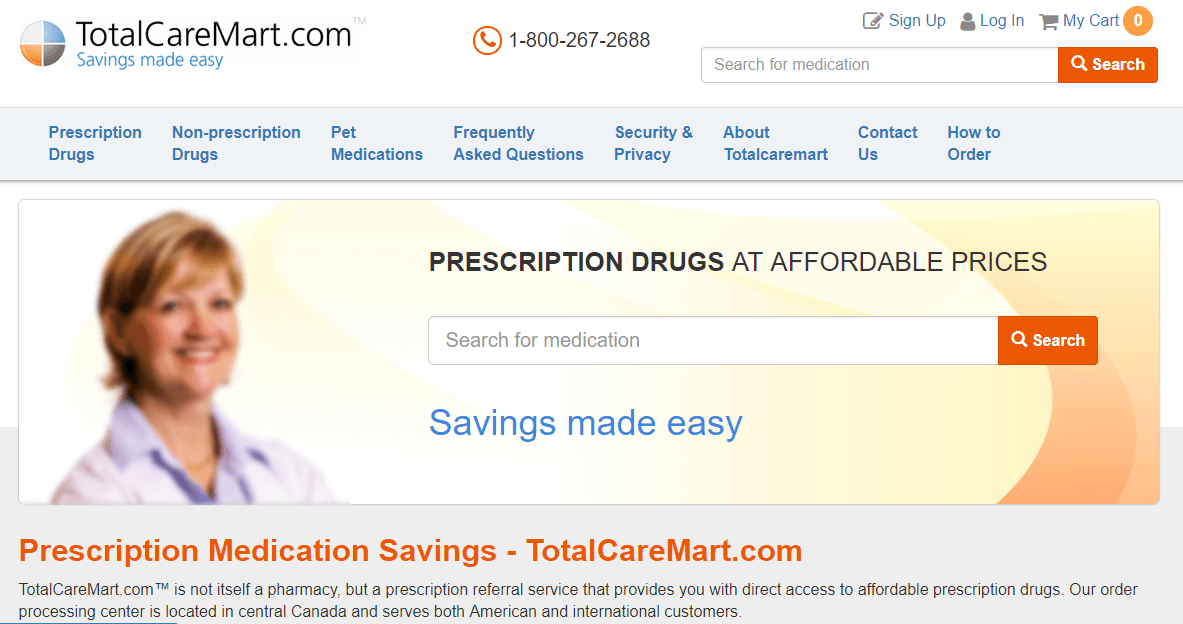A promotional banner for TotalCareMart.com features a blue and white background with various accents in orange and black. At the top of the banner, the orange text reads "Prescription Medication Savings - TotalCareMart.com". Below this, a white search bar appears prominently, encouraging users to "search for medication” or other related terms. To the left of the search bar is the image of a woman, possibly representing customer service or a satisfied user.

The central part of the banner emphasizes the company's services and benefits, with black text declaring, "Prescription Drugs at Affordable Prices". There's a showcase of various service categories such as prescription drugs, non-prescription drugs, pet medications, security and privacy, and more. 

The bottom of the banner reiterates the company's domain, "TotalCareMart.com", accompanied by their contact number, 1-800-267-2688. An additional note highlights their broad service reach: "Our order processing center is located in central Canada, serving both American and international customers."

Overall, the banner conveys TotalCareMart.com's commitment to providing affordable medication with efficient service, wrapped in a visually appealing layout of blue, white, and orange hues.